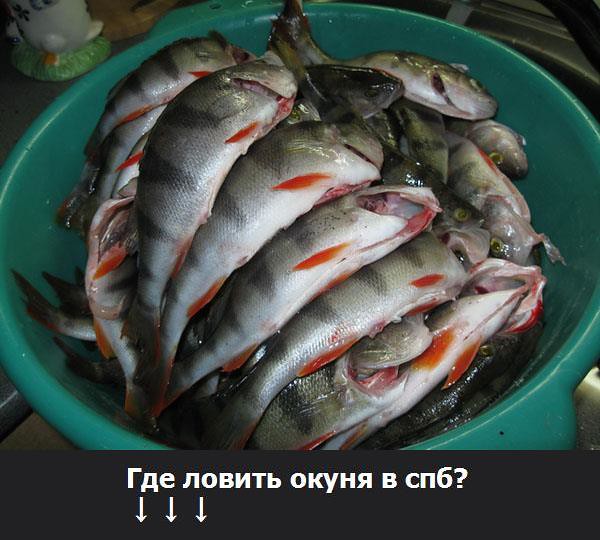The image portrays a tightly focused view of a blue-green plastic bowl filled with at least 20 to 30 cleaned and gutted fish, which have their heads, tails, and bright red fins intact. The fish exhibit a striking pattern of dark gray vertical stripes on their gray bodies, with a wet and slimy appearance. The fish are arranged with their tails predominantly on the lower left and heads on the upper right, creating a bulging effect due to their stacking. A strip at the bottom part of the photograph displays white Cyrillic text on a dark gray background with a question mark at the end, and three white downwards-pointing arrows on the left. The background is mostly obscured, with just a hint of some indistinct ceramic items on the tabletop.